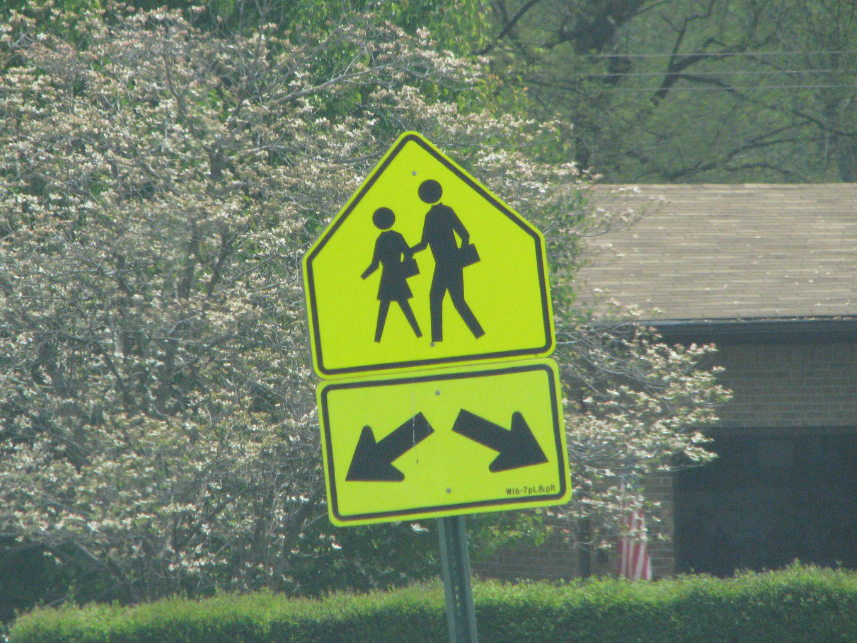This outdoor daytime image prominently features a street crossing sign mounted on a metallic pole structure in the middle. The sign consists of two parts: the top portion shaped like a house, depicting two people with circular heads carrying briefcases in their left hands and walking to the left, and the bottom rectangular portion with a bright yellow background, a black border, and two black arrows pointing diagonally downward to the left and right. In the background, a sprawling tree adorned with white flowers is visible, alongside a brick house with brownish-orange walls and a lighter brown rooftop. Hanging in front of the house is an American flag. Adjacent to the house, there's an open garage with a brown door, and a neatly trimmed hedge is in the vicinity. The image captures the serene atmosphere of a suburban setting with a blend of natural and constructed elements.